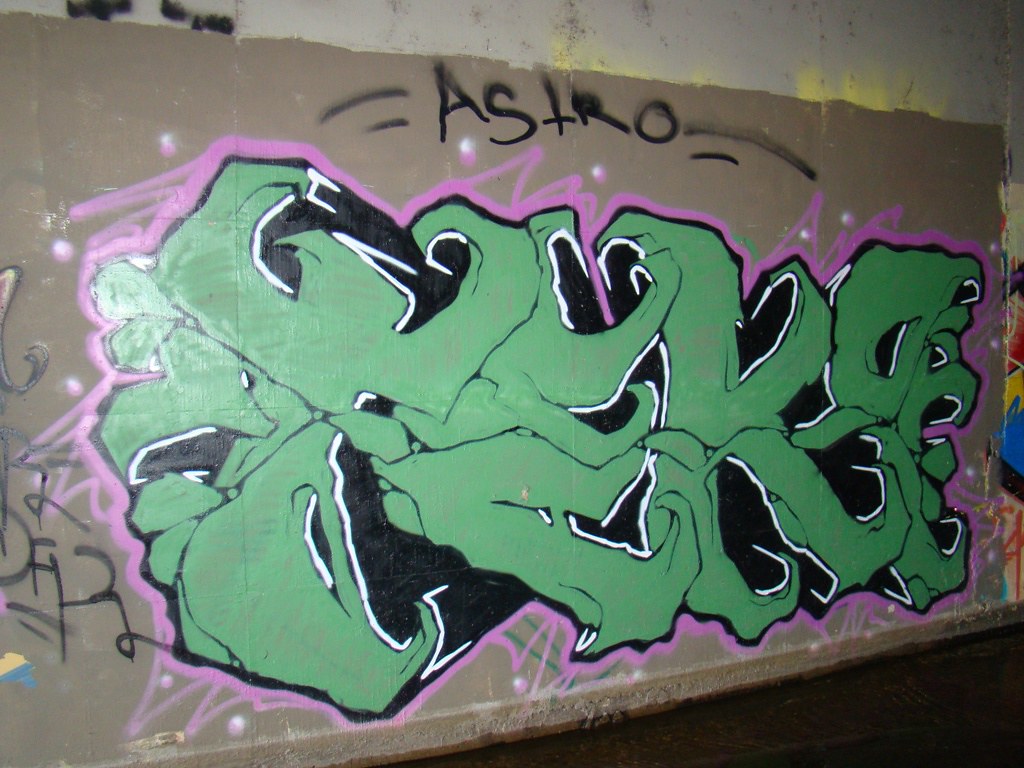The photograph captures a segment of a concrete wall, evidently part of an abandoned or poorly maintained building, characterized by accumulated dirt and signs of wear. The wall's material is concrete, with a portion conspicuously painted brown. On this brown section, the word "ASTRO" is spray-painted in bold black letters at the top. Beneath this, a heavily stylized green graffiti design dominates the composition, designed with such complexity that the letters become nearly indecipherable. This green text is detailed with black borders and intricate white lines, and a vivid pink outline encircles the entire green design, adding to its striking appearance. Evidence of multiple layers of paint, including hints of blue, yellow, and red graffiti covered by the brown paint, suggests repeated attempts to overwrite previous markings. Various additional lines and marks from markers are scattered around, further indicating the wall's extensive history of being a canvas for different artists. The overall color scheme of the concrete wall transitions from a lighter brown upwards to darker shades at the base, with no individuals present in the photograph. The frame of the image is slightly wider than it is tall, emphasizing the breadth of this richly textured and graffitied surface.